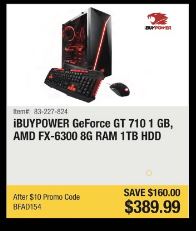The image features a black border with a creature depicted in the top right corner, its jaws open and fangs visible. In the center, there is a black PC case illuminated with red lights, accompanied by a black keyboard with red keys and a black mouse. The background is predominantly white. An "X" indicates item number 23227824. A gray square details the specifications: "iBUYPOWER, GeForce GT 710 1GB, AMD FX-6300, 8GB of RAM, 1TB HDD." Adjacent, a yellow rectangle advertises a promotional offer: "After $10 promo code V50154, save $160, $399.97." The message concludes with a "Thank you for watching."